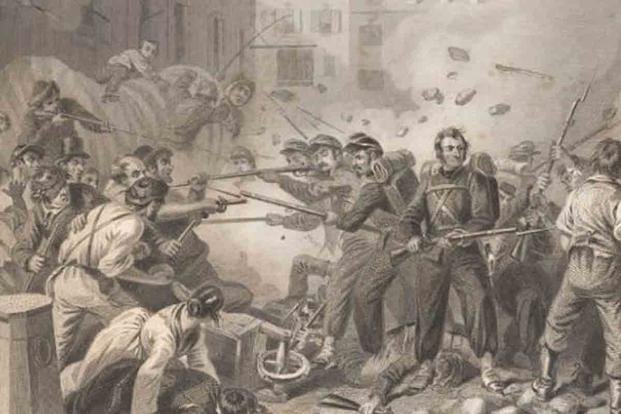The image appears to be a detailed painting or drawing, possibly from the early 19th century, depicting a chaotic battle scene in shades of black, white, and gray. In the foreground to the left, two women are prominently shown; one woman is shielding another, both ducking away from the ongoing skirmish. The scene is filled with men wielding rifles with bayonets, indicating an intense conflict. The soldiers on the right are wearing darker uniforms and seem more organized, while those on the left appear to be civilians, some in top hats, possibly engaged in a revolt or protest. In the upper left corner, a child is perched atop a statue or creature, adding to the tumultuous atmosphere, which also features debris and an overturned cart. The piece, rendered in a style resembling charcoal or pencil, captures the frenzied and violent nature of the clash.